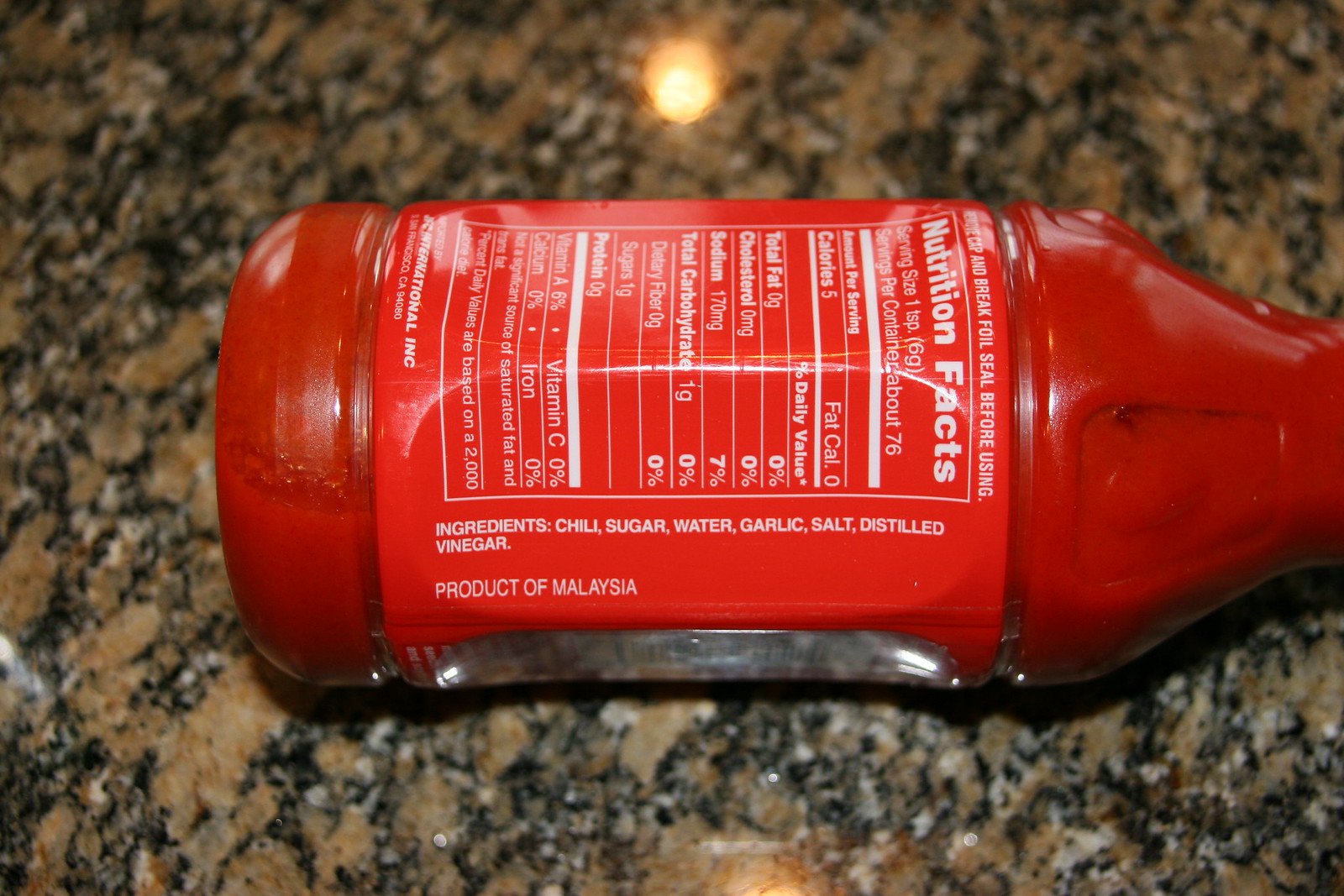This close-up photograph features an overturned cylindrical glass bottle of red chili sauce lying horizontally on a chocolate brown marble countertop with specks of black, white, and light gray. The sauce appears almost like a puree, contained within a bottle wrapped in a red label with white text. The label prominently displays nutritional information: serving size 1 tablespoon (6 grams), 76 servings per container with each serving providing 5 calories and no fat or cholesterol. It also shows 170 milligrams of sodium (7% of daily value), 1 gram of total carbohydrates, 1 gram of sugar, no dietary fiber or protein, and it includes 6% of daily vitamin A but no calcium, vitamin C, or iron. The ingredients listed on the label include chili, sugar, water, garlic, salt, and distilled vinegar, indicating the product is manufactured in Malaysia.